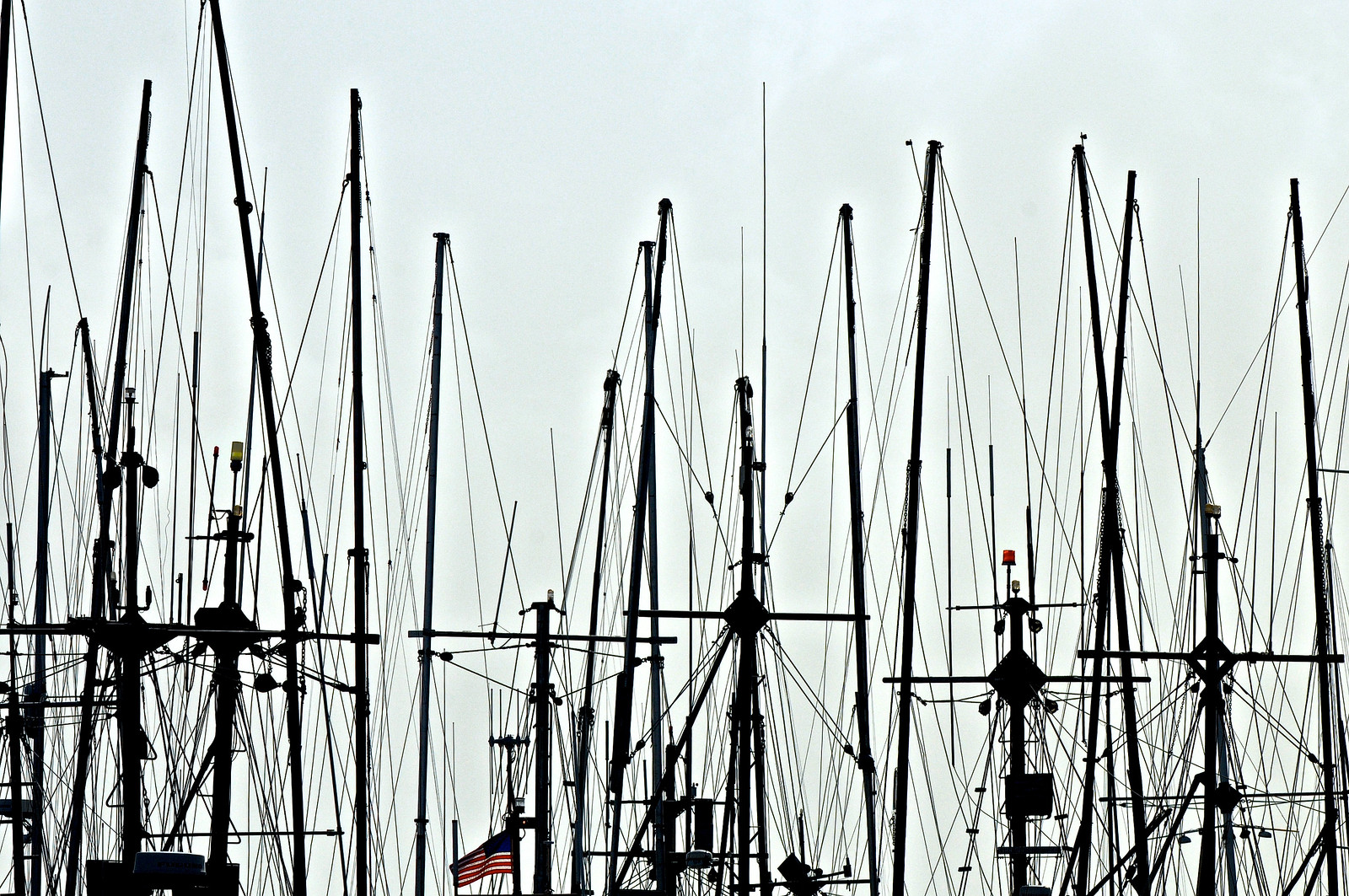This photograph captures the intricate and complex view of numerous sailboat masts and possible radio antennas. Taken from an elevated perspective, the shot focuses solely on the upper portions of these vessels, presenting a dense forest of masts, poles, and wires crisscrossing in every direction. The scene is set against a pale blue sky with faint wisps of white clouds, giving it an overcast appearance. Each mast is equipped with a network of ropes and wires, some of which appear as silhouettes due to the angle of the light. The structures are so elaborate that they likely belong to large, sophisticated sailboats. An American flag can be seen toward the bottom middle of the frame, fluttering near one of the central masts. The overall image evokes a sense of organized chaos with its tangle of lines and rigs, highlighting the complexity and grandeur of maritime craftsmanship.